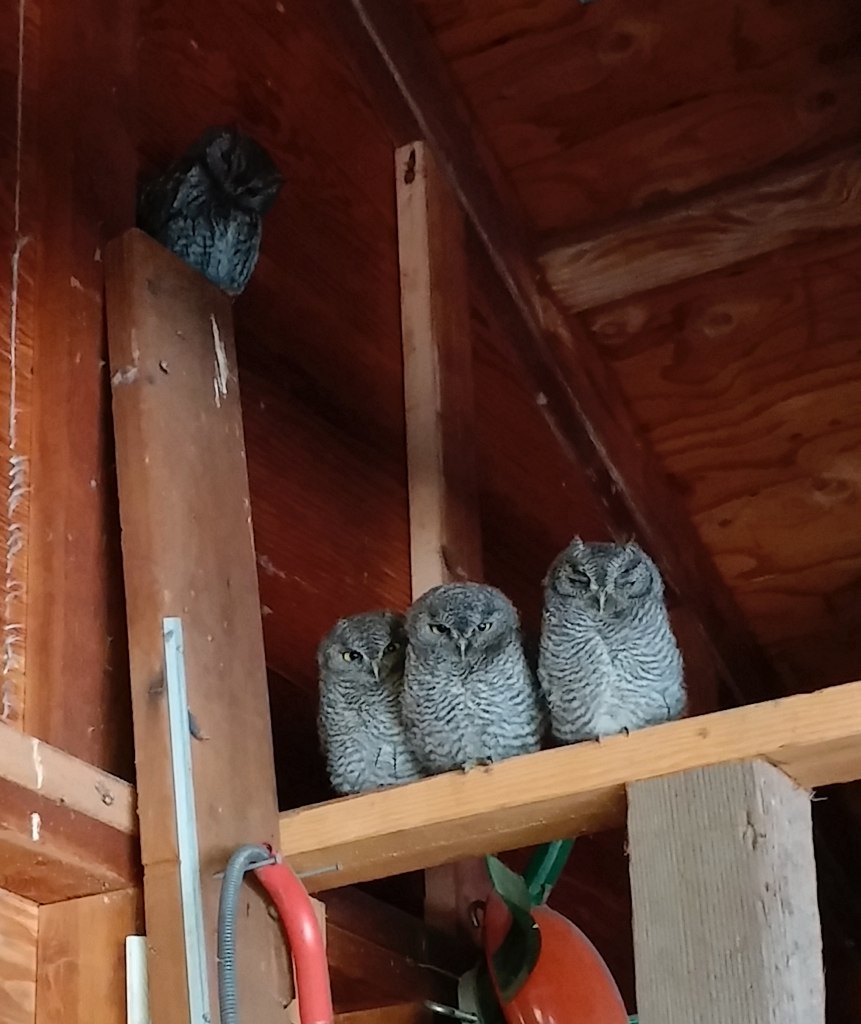The image is a color photograph taken inside what appears to be a barn or shed, showcasing the intricate wood construction in a portrait orientation. Various types of wood frame the structure: the ceiling features a dark cherry red, varnished wood, while the foreground includes a horizontal plank of a warm pine color supported by a vertical, grey ash-toned upright. Dominating the center of the scene, just below the horizontal middle, three owls perch side by side on the pine plank, facing the camera. Each owl displays zebra-like black and white stripes radiating from a central line on their bodies, with slightly darker grey to black faces. Another owl, partly in shadow, perches high on a separate vertical plank against the left side. This fourth owl appears darker, possibly due to the lighting. Additional details include a red object with a black pipe hanging lower in the image, and a green and red object on the bottom right side. The composition encapsulates the rustic ambiance of the shelter and the mesmerizing presence of the owls.